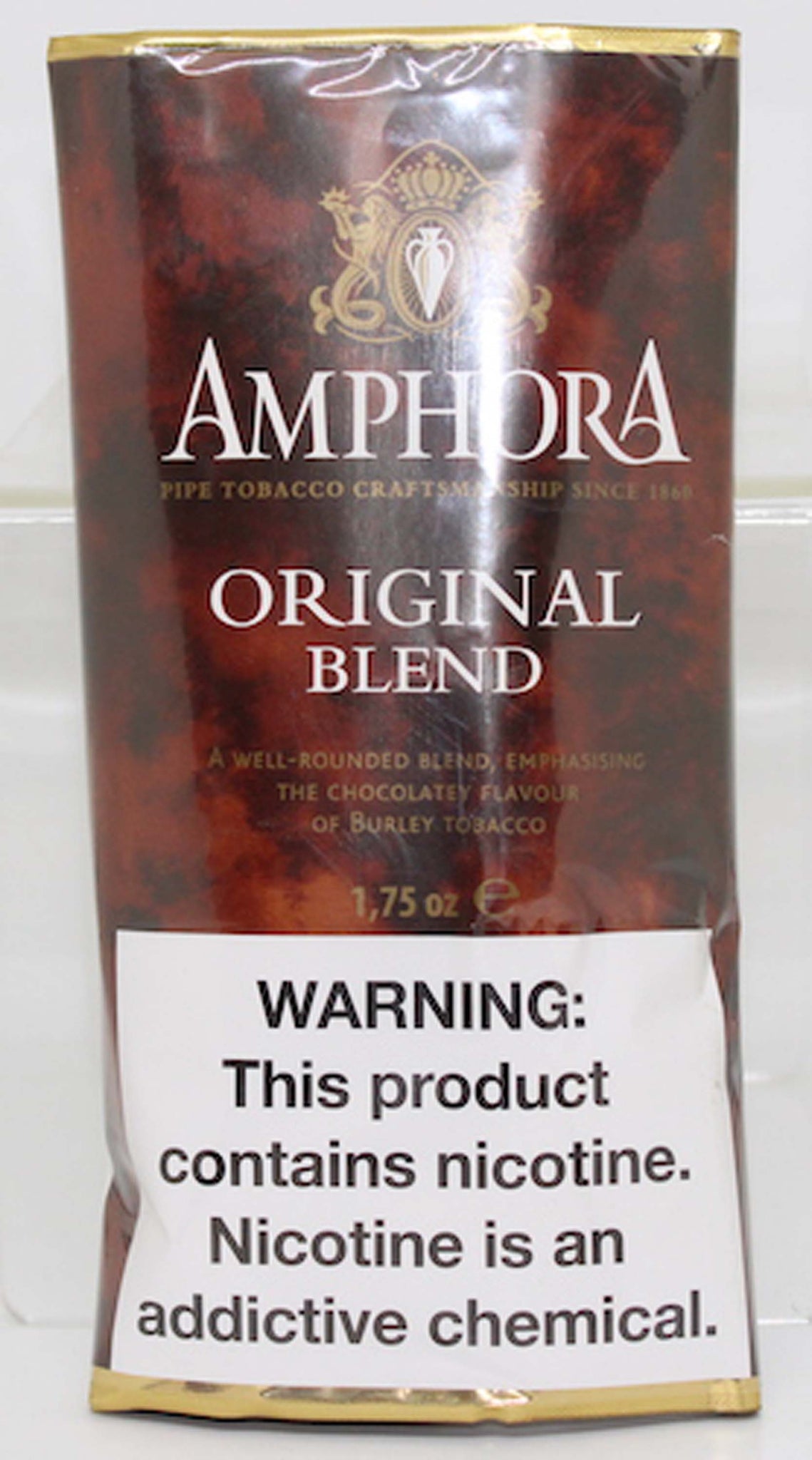The photograph features a predominantly maroon and crimson marbleized package of Amphora tobacco, positioned against a white porcelain tile. The top and bottom of the package are trimmed with gold, and at the top is the Amphora logo, featuring two mermaids and a crown. In large, capitalized white text, it reads "AMPHORA," with "Pipe Tobacco Craftsmanship" in smaller gold capitals below it, suggesting it dates back to 1849, though the exact year is partially obscured. "Original Blend" is emblazoned in bold, capitalized white text beneath that, followed by a description in smaller gold font that reads, "A well-rounded blend emphasizing the chocolatey flavor of Burley tobacco." The package contains 1.75 ounces of tobacco and prominently displays a white warning label with black text stating, "WARNING: This product contains nicotine. Nicotine is an addictive chemical."